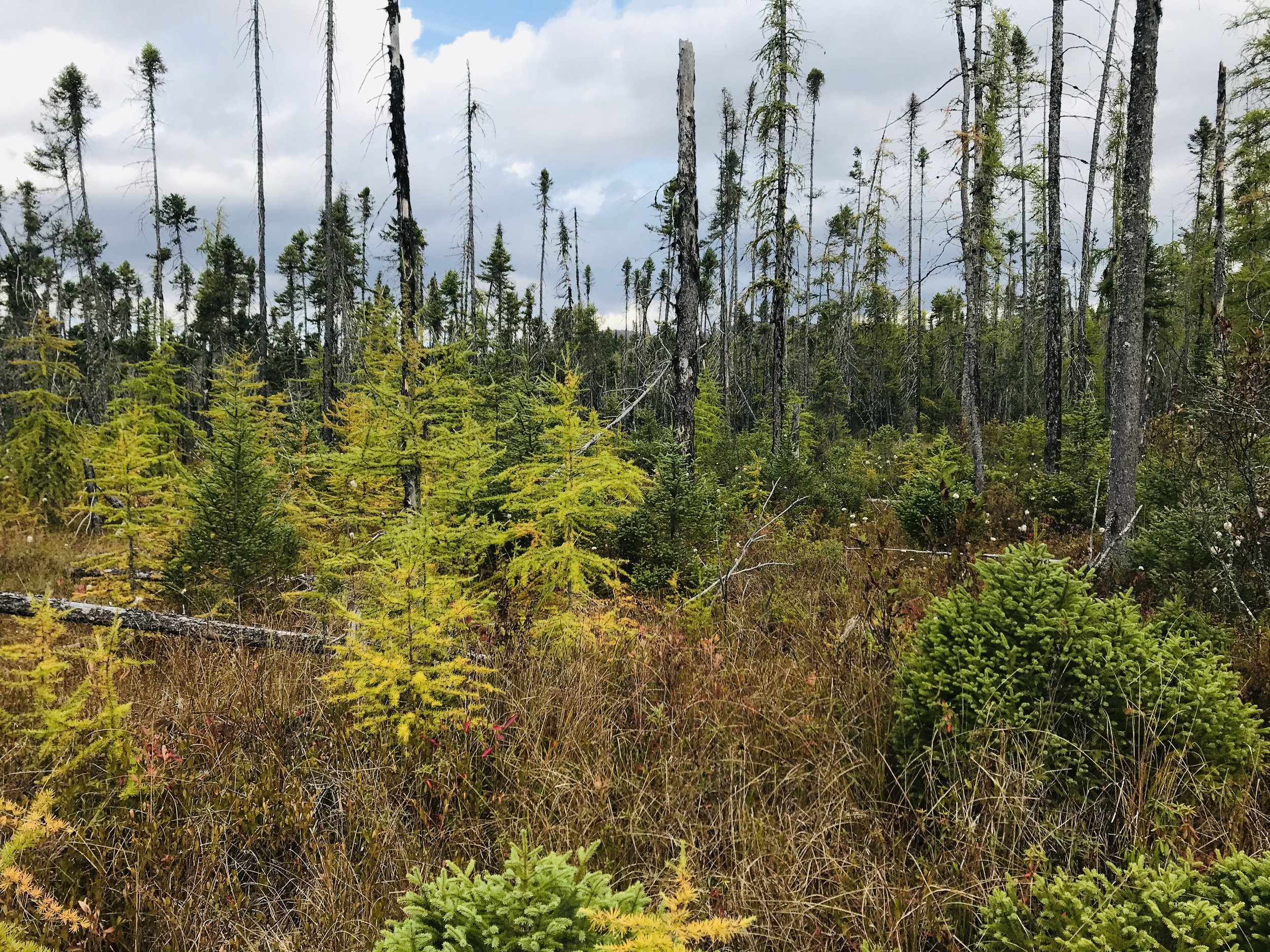This horizontal landscape photograph captures a sparse forest seemingly affected by fire or recent deforestation. The upper one-third of the image displays a sky predominantly covered by fluffy white and gray clouds with only small patches of blue peeking through. The lower portion features tall, overgrown tan grass interspersed with saplings and new growth, mostly consisting of evergreen trees. These saplings vary in color from light green to yellowish tones, with a few displaying darker green hues. 

In contrast, the middle of the image is dominated by taller, barren trees with limbless stumps and bare trunks, some showing new growth at their tops, suggesting fire damage. The ground beneath these taller trees is littered with dead or partially dead foliage and plants, adding a brown and lifeless appearance to the scene. A mix of green, brown, and yellow vegetation covers the area, adding to the sense of desolation. 

Towards the background, fuller trees with more greenery are visible, indicating that this affected area may be part of a larger, recovering forest. The absence of people or animals further emphasizes the quiet and stillness of this regenerating landscape.